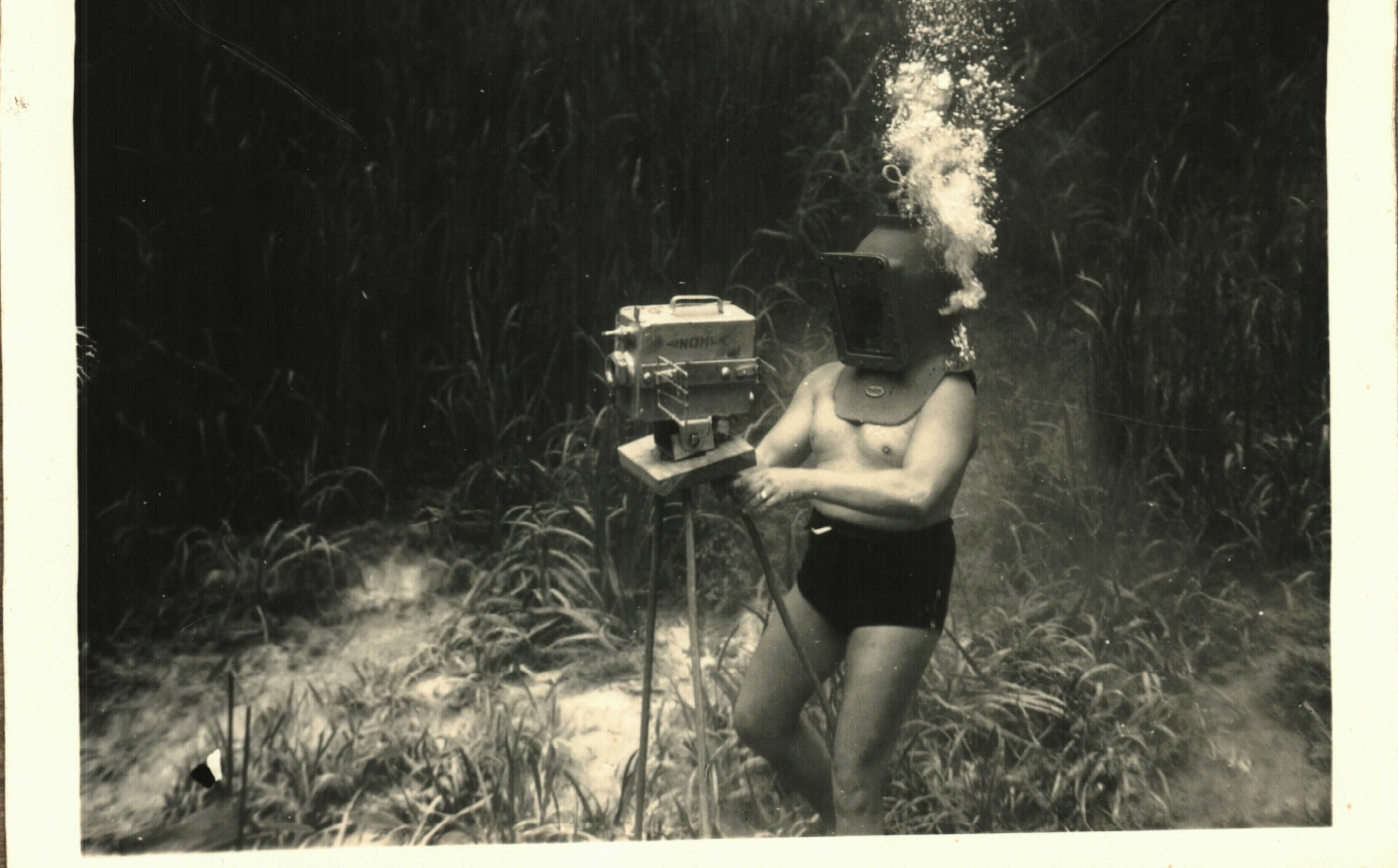This is a detailed black-and-white photograph of a shirtless man underwater, wearing dark swim trunks and an old-fashioned diving helmet with an attached breathing apparatus. Air bubbles are visibly rising from the helmet. The man is operating an underwater camera mounted on a tripod, with a white border around the image indicating its vintage nature. The seafloor in the background is covered in seagrass, some of which appears taller than the man himself. The scene is relatively deep, estimated between 15 to 45 feet, and devoid of any noticeable fish or other people. The overall image is clear and well-lit, despite the depth, capturing the detailed textures and elements of the underwater environment. A wedding ring on the man's finger adds a personal touch to the historical and professional feel of the photograph.